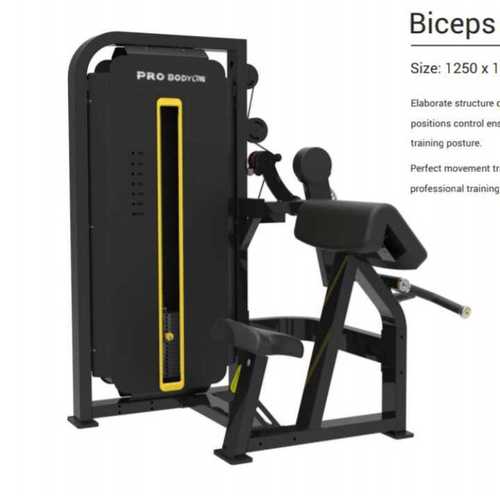The image depicts a sophisticated bicep workout machine prominently branded as ProBodyOn, situated against a plain white background. The machine is predominantly black with distinctive yellow accents, particularly on the section that houses the weights. The ProBodyOn label appears clearly on the top part of this weight section. The machine's design features an elaborate structure aimed at providing optimal training posture and controlled movements, ensuring a perfect workout specifically for the biceps.

Key text accompanying the image, though partially cut off, reads: "BICEPS, size 1250 x 1." Further readable phrases include, "elaborate structure, positions control, training posture, perfect movement, professional training," which emphasize the machine's focus on precision and effectiveness in bicep exercises. The equipment also incorporates metal bars and wires connecting various parts, including a seating section with an armrest, suggesting a well-integrated system for targeted bicep training. The meticulous design hints at a highly engineered product ideal for professional-grade workouts.